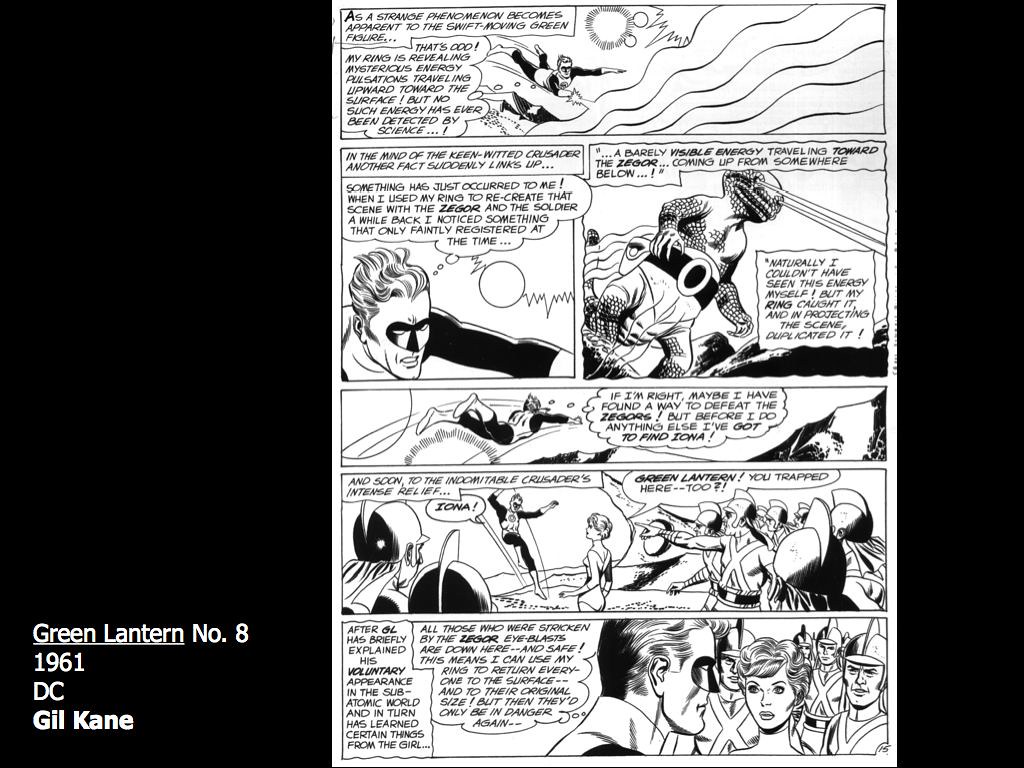This image is a detailed black-and-white comic book page from *Green Lantern* No. 8, published in 1961 by D.C., illustrated by Gil Kane. The page features a large black border on both the left and right sides, with white text at the bottom left corner stating "Green Lantern, No. 8, 1961, DC, Gil Kane." 

The page consists of six panels in five rows. The top panel is a single wide box with extensive text along its left side, setting the scene as the Green Lantern notices a strange phenomenon. Below that, the second row contains two narrower panels side by side, continuing the narrative with more dialogue-heavy scenes. 

The remaining three rows each contain a single panel. The action-filled illustrations depict the Green Lantern battling what appears to be a giant creature, reminiscent of Godzilla. Additionally, there are characters who seem to be soldiers, with X-shaped suspenders and helmet-like headgear that resemble Spartan helmets. Various human faces, both men and women, add to the complexity and detail of the scene, suggesting a multifaceted plot with multiple characters and interactions.